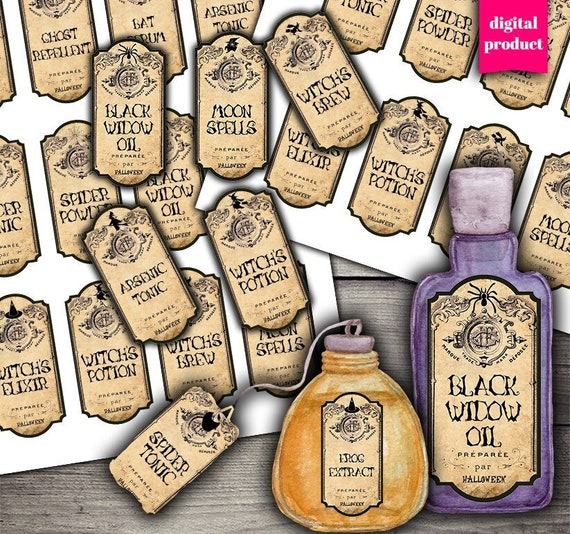This image is a digital illustration depicting various Halloween and witch-themed products, likely for printable labels. Dominating the picture is a black wheel labeled "Black Widow Oil," accompanied by a pink ribbon in the top right corner that reads "Digital Product." At the bottom right, there are two bottles; the first is a small orange bottle labeled "Frog Extract" with a witch's symbol, and the second is a larger purple bottle labeled "Black Widow Oil" featuring a spider and another logo. The image also contains various wooden tags with product names such as Moon Spells, Witch's Brew, Arsenic Tonic, Witch's Potion, and Spider Tonic. The labels are detailed with intricate designs, signifying their decorative and seasonal nature. This appears to be an advertisement for purchaseable, printable labels, ideal for creating festive Halloween decorations.